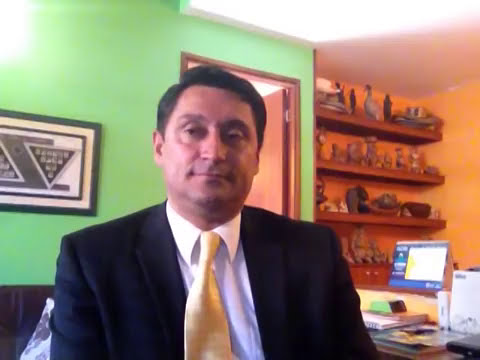The image features a middle-aged man in his 40s, with black hair, smirking subtly rather than fully smiling. He is dressed in a black sports coat, a white button-up shirt, and a yellow tie, and is seated at a desk. Behind him, to the left, the wall is painted lime green and adorned with a picture that includes a gray backward "Z" and a barely readable yield sign. To the right of the man, the foreground shows a cluttered desk featuring a computer monitor and an assortment of books. The background includes an orange wall to the upper right, where four wooden shelves are mounted. These shelves are populated with various wooden objects including ducks, tiki figures, and possibly Buddha statues.